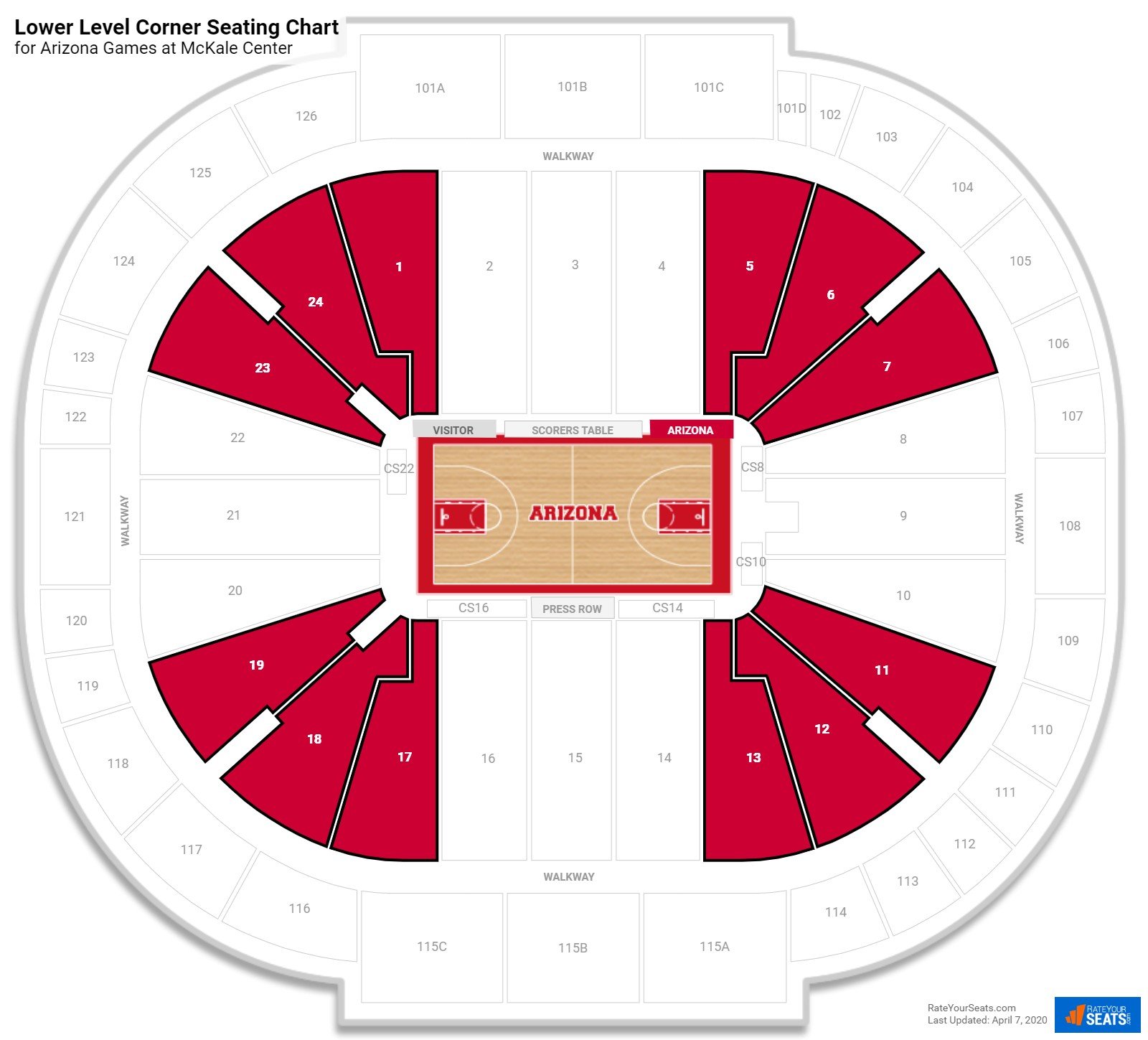This detailed seating chart provides an overview of the Lower Level Corner Seating at McKale Center for Arizona games. Dominantly featuring a circular design, the chart prominently displays rows of seats encircling the court area in hues of white, gray, and red. 

At the top of the image, sections are labeled 101A, 101B, and 101C, with numbers extending outward. Likewise, the bottom portions show sections 115C, 115B, and 115A. Central to the image are seating banks colored in red and white, each meticulously numbered. A noticeable pop-up box highlights the visitor’s area along with the scores table. 

The center court, colored tan and adorned with 'ARIZONA' written in bold red letters, features basketball hoops at either end. Surrounding the court, the seating areas are marked with an array of letters and numbers. 

Furthermore, at the bottom of the chart, a white, blue, and orange box stands out, accompanied by gray font indicating the chart was last updated on April 7th, 2020.